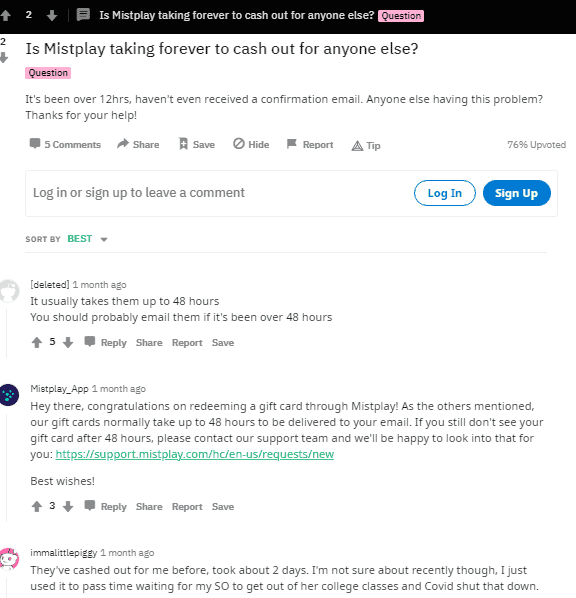Here is a detailed and cleaned-up caption for the image:

"Set against a white background, the screenshot features a black header with white text that reads, 'Is Misplay taking forever to cash out for anyone else?' To the right of this, a pink box labeled 'Question' is visible. Below, on the white background, the same question is reiterated: 'Is Misplay taking forever to cash out for anyone else? It's been over 12 hours and I haven't even received a confirmation email. Anyone else having this problem?' Beneath this text, it shows '5 comments' and '76% upvoted.' A box prompts users to 'Login or Sign Up to leave a comment,' with two buttons to the right: a white one with a blue border labeled 'Login' and a blue button with white text labeled 'Sign Up.' Below this prompt, it says 'Sort By Best' in green text with a pull-down arrow. The first response reads, 'It usually takes them up to 48 hours. You should probably email them if it's been over 48 hours,' accompanied by an upvote count of five."